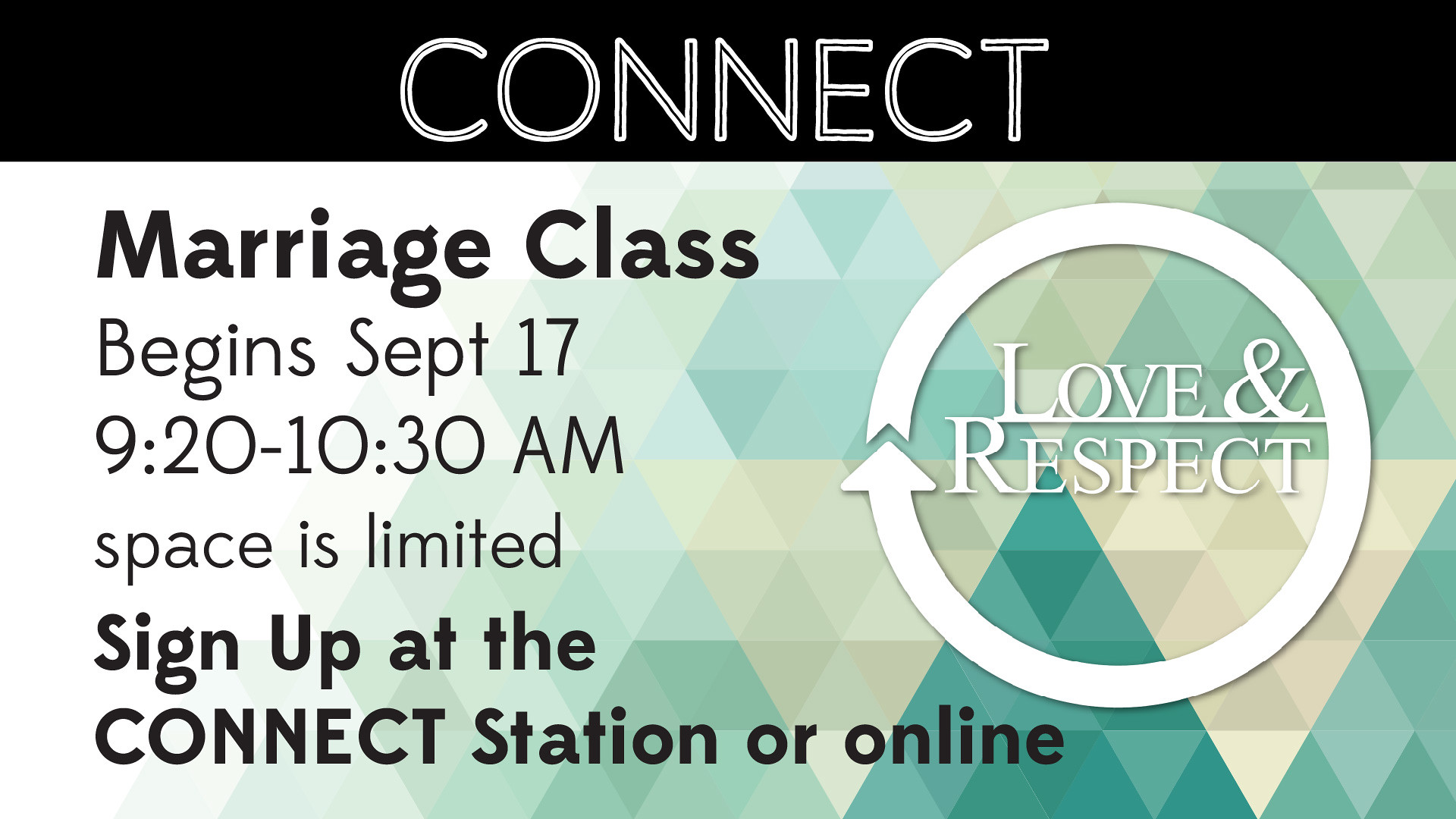The advertisement showcases a marriage class set against a fractal-like background composed of various shaded triangles in greens, yellows, darker greens, and hints of blue. Dominating the top of the image is a black banner with the word "CONNECT" written in bold black text outlined in white. Below this, the main details of the event are displayed in black text: "MARRIAGE CLASS BEGINS SEPTEMBER 17, 9:20 to 10:30 AM. SPACE IS LIMITED. SIGN UP AT CONNECT STATION OR ONLINE." On the right side, there's a white circular emblem designed as an arrow looping back on itself, enclosing the words "LOVE and RESPECT" in white text. The cohesive color scheme and clean geometric background lend a modern and organized aesthetic, clearly designed to draw attention to the class details.